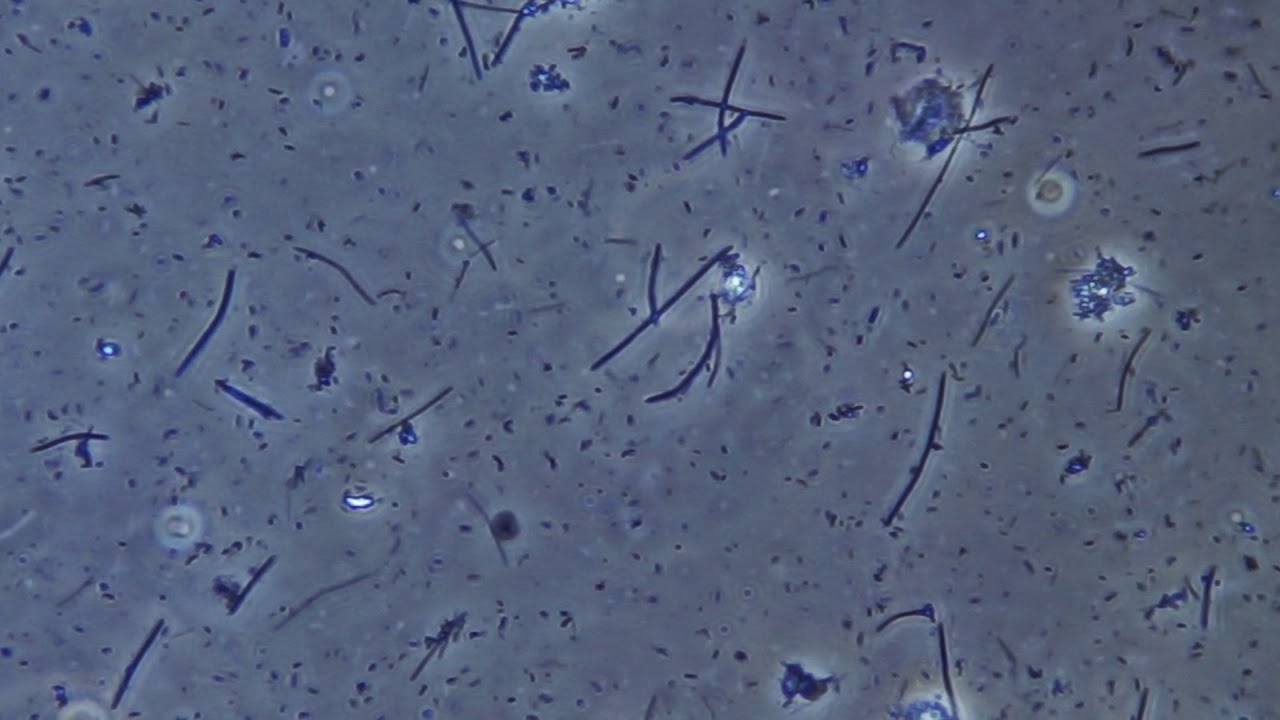The image appears to be a highly detailed, microscopic view of various microbial organisms or molecules, predominantly tinted in shades of blue, gray, and white. The entire scene is filled with dozens of tiny structures, including both stick-like and circular forms, with darker shades of blue indicating larger organisms and lighter shades suggesting those closer to water or more transparent areas. The background and overall tone are bluish-gray, giving the image a somewhat gloomy appearance. Among the myriad of microscopic entities, some resemble tiny seeds or grains of rice, while others resemble pine needles, often overlapping and scattered across the slide. Additionally, there are brighter clumps and spiky formations illuminated with lighter blue and white hues. A variety of small, circular dots with glowing lighter edges add to the intricate and textured composition.